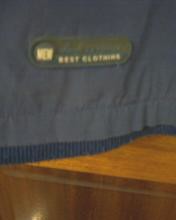A detailed description of the photograph could be:

"The image captures a piece of light blue fabric spread across a wooden table. The fabric is visibly wrinkled and bunched, with noticeable ridges at the bottom. At the center of the fabric, there is a circular green object. To the left side of this object, the word 'NEW' is clearly printed in white letters. In the bottom right corner, a partially visible text reads 'something clothing,' suggesting it could be part of a larger label or tag. The fabric appears to be finely stitched, with several folds and curves, especially towards the bottom where it curves inward and then extends to the right. The wooden table underneath is light brown, complementing the warm tones of the light wood wall seen in the background. A faint, grainy patch of light is visible in the bottom left corner of the image, illuminating the fabric and adding depth to the scene."